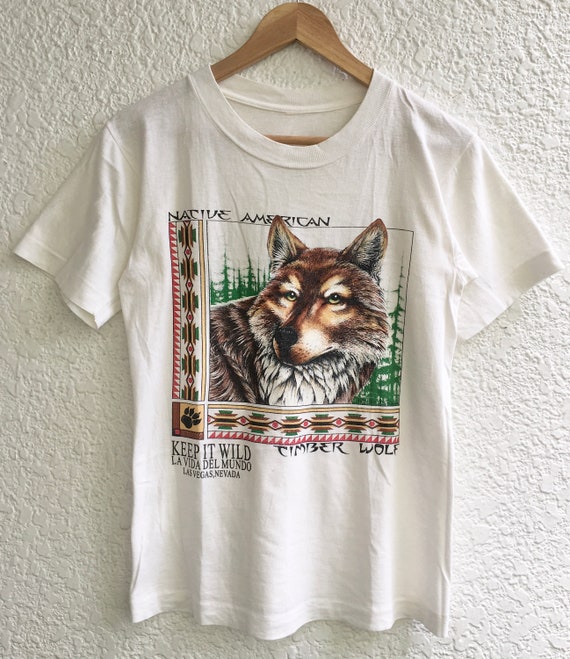The photograph features a wrinkled, off-white crew neck t-shirt hanging on a quality brown wooden hanger against a cream-colored stucco wall. Centered on the front of the t-shirt is a square image depicting a brown wolf with piercing green eyes surrounded by green trees. Above the wolf, in bold black letters, it reads "Native American." Below the image in the lower right corner, it says "Timber Wolf," while in the lower left, it states "Keep it Wild La Vida Del Mundo, Las Vegas, Nevada." Framing the image is a striking Native American print in shades of green, cream, black, and red. The detailed design, along with the vibrant print and balanced text, all highlight the t-shirt's central theme of nature and cultural appreciation.